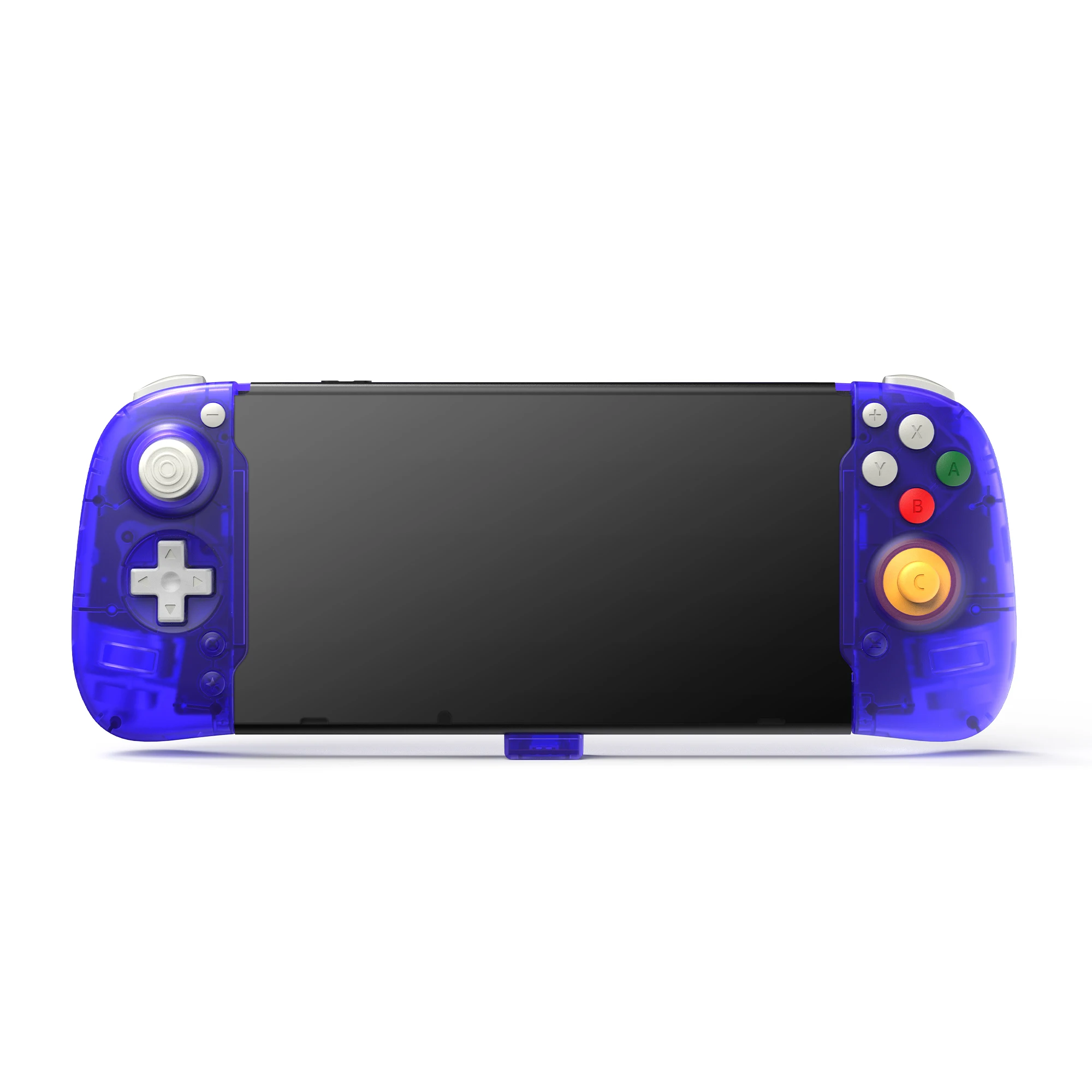The image showcases a handheld Nintendo gaming console that appears to be a customized Nintendo Switch. The central part of the device features a large black screen. The sides of the console are adorned with transparent blue, almost semi-circular, detachable joy-cons that emulate the classic GameCube controller design. On the left side of the console, the joy-con includes a gray joystick at the top left and a directional pad with the classic up, down, left, and right arrows below. The right joy-con houses the X, Y, A, and B buttons with distinct colors: A is green, B is red, while the X and Y buttons retain a neutral shade. Below these buttons, there is a yellow joystick labeled with the letter C. Both joy-cons reveal their internal circuitry through the translucent blue plastic. The resemblance to the GameCube controller layout is evident with these custom modifications, including the joystick positions and button colors, offering a retro aesthetic blending older and newer Nintendo designs.